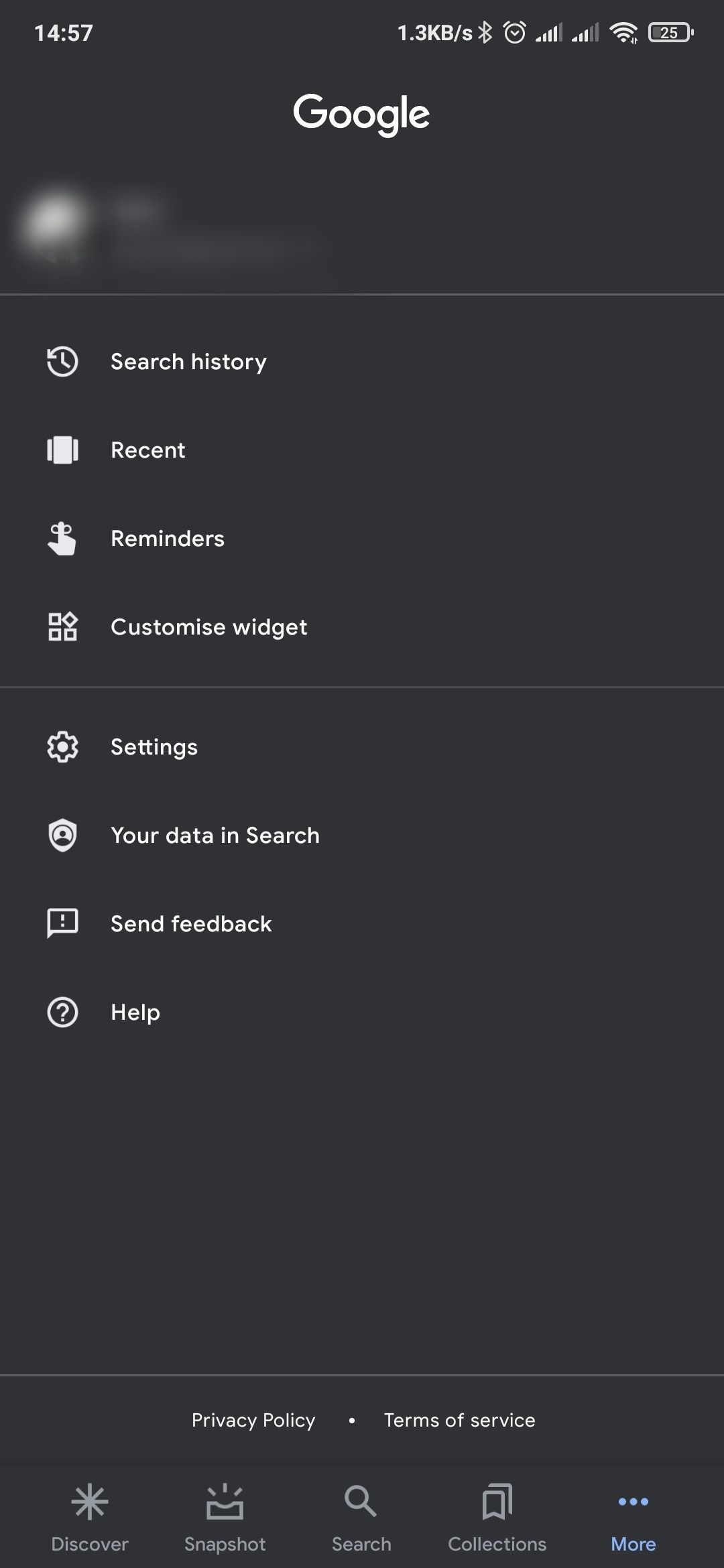This is a mobile screenshot taken from a Google device or Google app display. The interface is set in dark mode, with a predominantly black background and white text, except for the 'More' icon, which is highlighted in light blue at the bottom right corner. The top section features the Google logo, with the user's profile picture and name blurred out for privacy. Below this, several options are visible: 'Search History,' 'Recent Reminders,' 'Customized Widget Settings,' 'Your Data in Search,' 'Send Feedback,' and 'Help.' At the bottom of the screen, there are links to the 'Privacy Policy' and 'Terms of Service.' Furthermore, a navigation bar at the very bottom showcases five icons: the 'Discover' icon, 'Snapshot' icon, 'Search' icon, 'Collections' icon, and a triple-dot 'More' options icon. The screenshot captures the status indicators in the top right corner, showing cell service, Wi-Fi connection, battery percentage, and the time, which reads 14:57. This detailed and meticulously organized interface, alongside the status indicators, confirm that the screenshot was taken from a mobile phone.